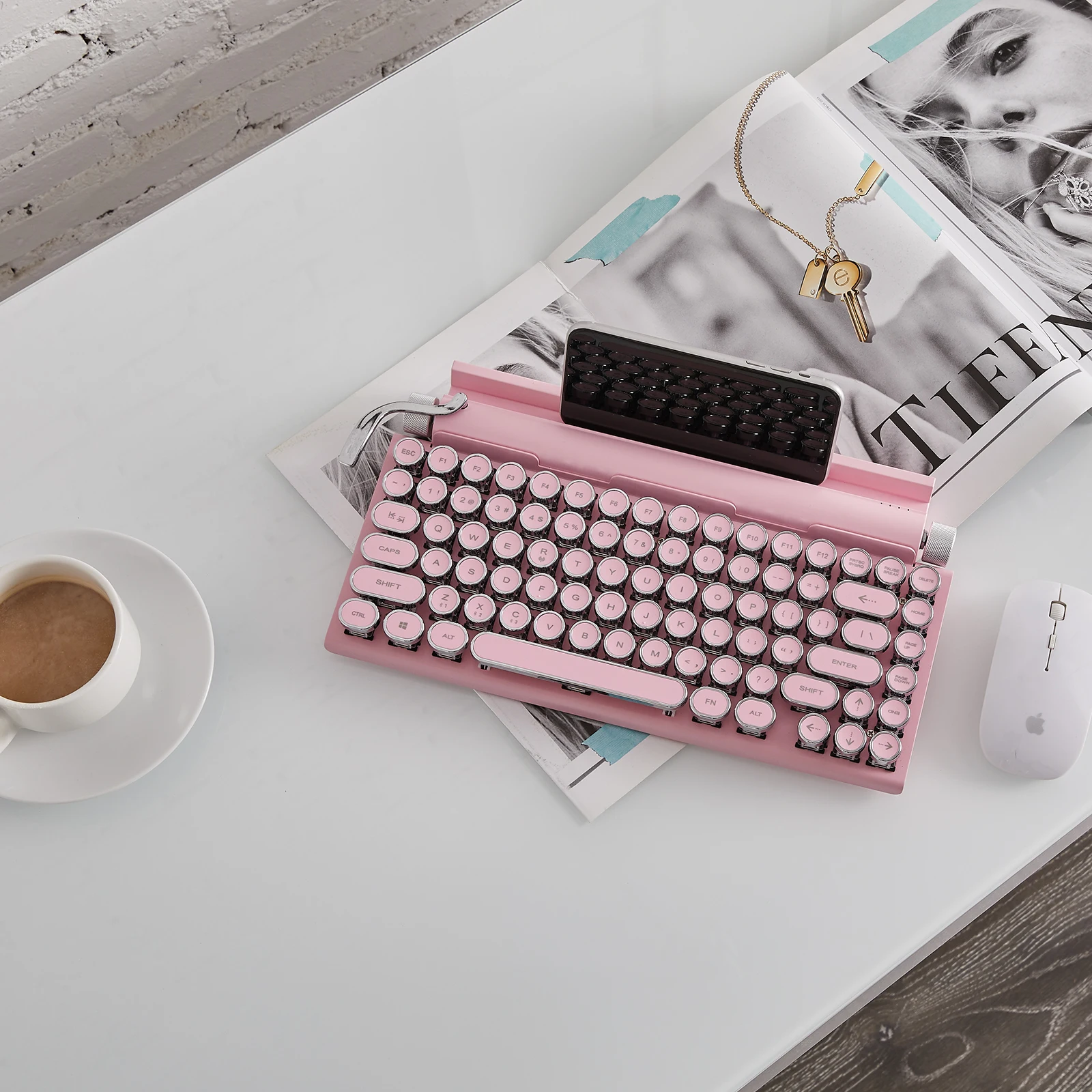The image displays a digital augmented reality photograph of a vintage-style typewriter keyboard designed for a smartphone, in a vibrant pink color with round and some oval keys. The keyboard is placed prominently on an open fashion magazine, resting on a white table surface. A smartphone acts as a screen, positioned horizontally in a holder where paper would normally emerge from a typewriter. To the right of the keyboard, a white Apple computer mouse is visible. On the left side of the table, there is a white cup of coffee with cream on a matching saucer, adding a cozy touch to the setup.